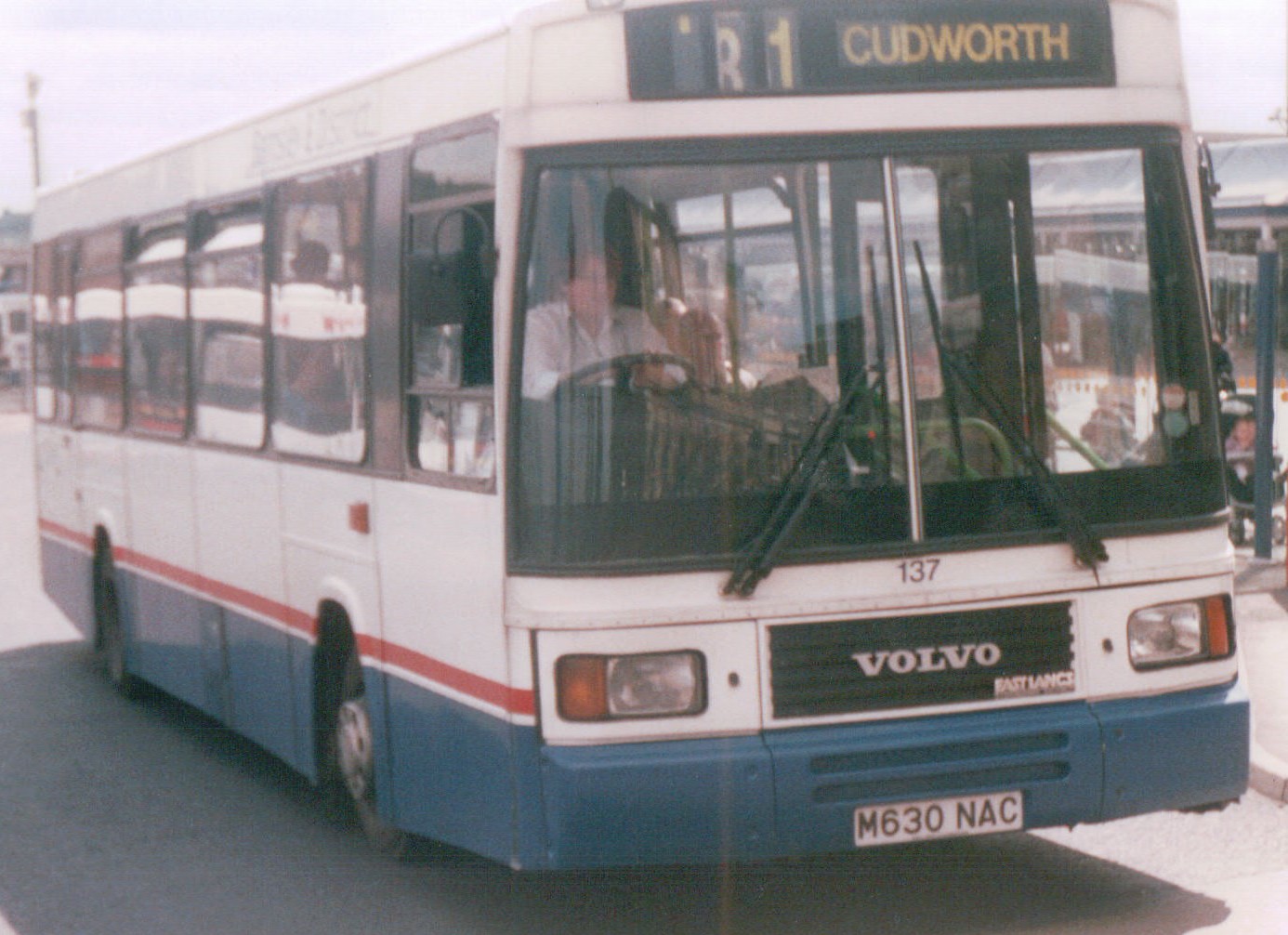The image showcases a front-facing view of a white Volvo bus with blue trim at the bottom and an orange stripe along the side. The license plate reads M630 NAC, and the destination displayed at the top is "818 Cudworth." This photograph is taken during the daytime under a clear blue sky, evidenced by the bright reflections on the side windows. The bus is operated by a female driver, seen wearing a white button-down shirt and glasses, steering the vehicle down a street. Adjacent to the bus is a curbside bus stop, identifiable by a waiting area with a canopy. A woman with a baby in a carriage is among the people waiting at the stop, suggesting the bus is about to pull in. In the backdrop, a light pole and a distant building can be observed, enhancing the urban setting of the scene. The inside of the bus appears to be green, and its fleet number is 137.